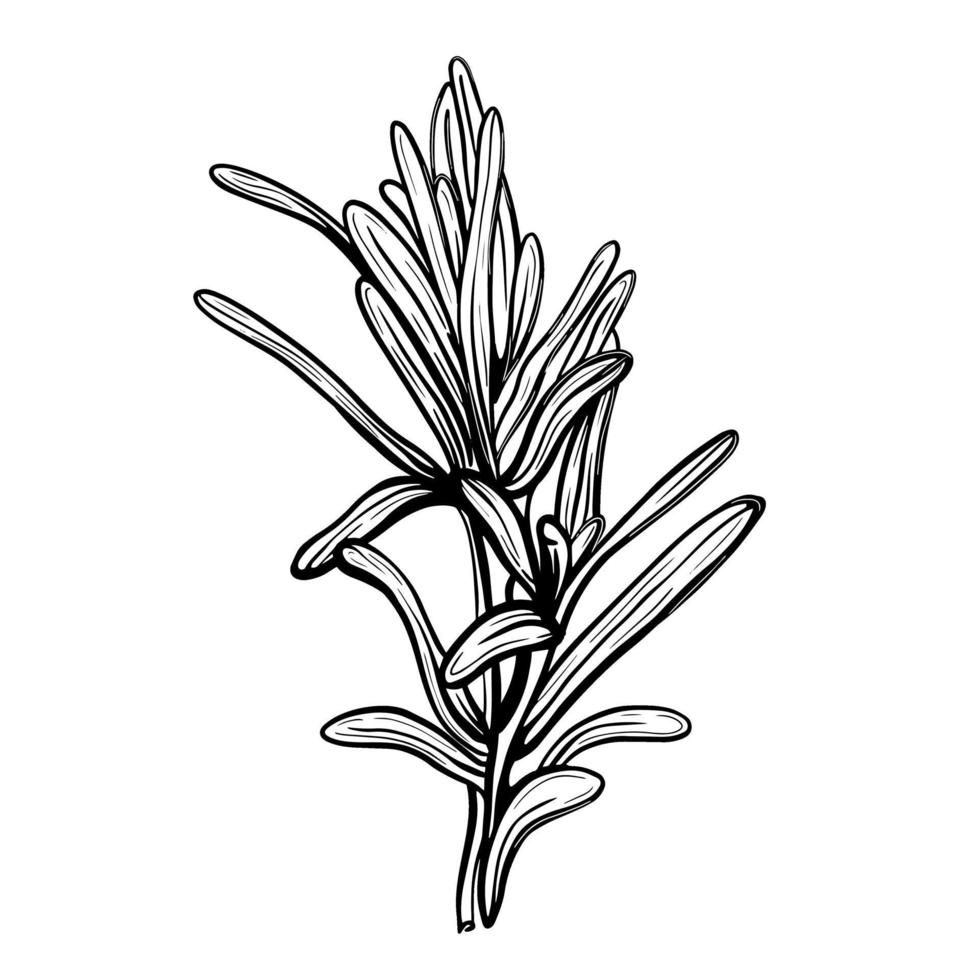The black-and-white image features a highly detailed drawing of a single rosemary plant, positioned upright at the center. The plant is illustrated with thick black outlines and thinner lines intricately detailing its numerous, narrow leaves. The rosemary's central stem branches into two sections, from which dozens of leaves jut out in various directions, creating a complex and textured appearance. The background and the plant itself are consistently rendered in pure white and true black, respectively, emphasizing stark contrast. The sketch gives the rosemary a lifelike quality as if it has been extracted from a natural setting or botanical book. There are no additional elements such as text, animals, or human figures, focusing the viewer's attention solely on the detailed structure and form of the plant.